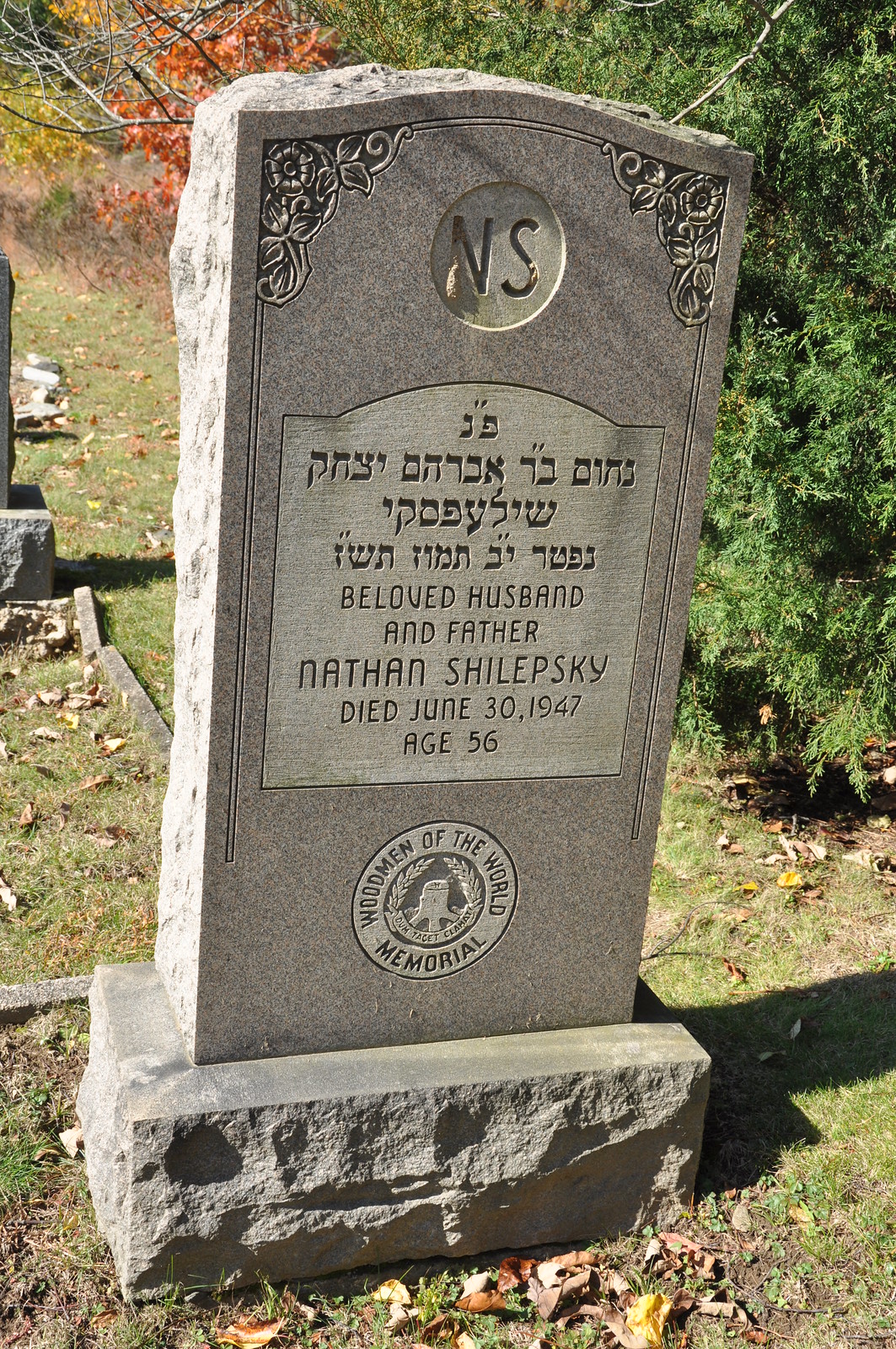The image features an ornate tombstone standing prominently in a cemetery, surrounded by green grass and autumn leaves, with trees providing a colorful backdrop. The headstone, approximately two to three feet tall, is intricately etched with flowers carved in the top corners and framed with elaborate borders. The initials "NS" are inscribed at the top, likely representing Nathan Schepelsky. Beneath the initials, there are a couple of lines of Hebrew text followed by an English inscription that reads, "Beloved Husband and Father Nathan Schepelsky, died June 30, 1947, age 56." At the bottom of the tombstone, a logo with the wording "Women of the World Memorial" is visible. Other headstones in the background confirm the setting as a peaceful cemetery.